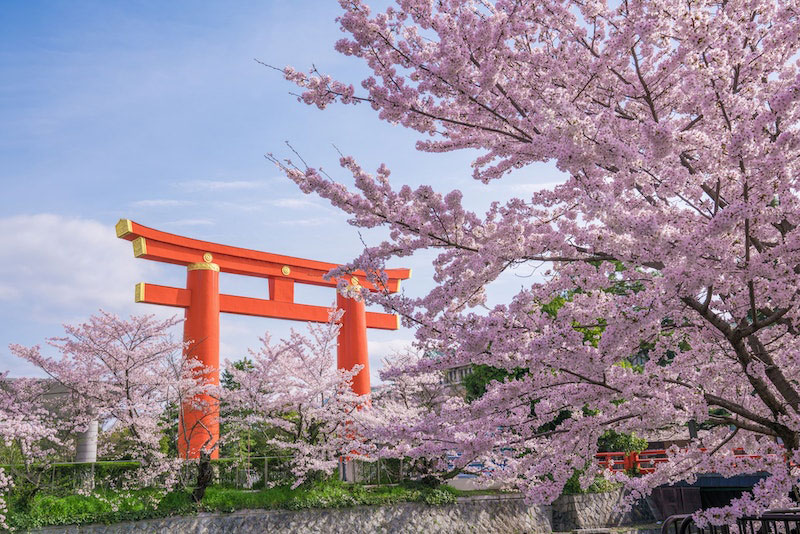The photograph is a detailed outdoor scene captured during daytime, featuring a prominent Shrine Gate on the left side, predominantly red with touches of gold. The gate is supported by two wide, round posts and has horizontal crossbars with yellow details. The gate is situated in a lush garden adorned with a variety of plants.

On the right side of the image, you find a large tree, possibly a lilac or cherry blossom, boasting a profusion of light pink to lavender flowers. There are more of these flowering trees scattered throughout the background, with their branches full of vibrant blooms. Visible through the opening in the trees is an orange fence-like structure, which may be part of the shrine's surrounding area. The lower part of the image has what appears to be a white wall, adding to the structured elements within the natural setting.

The sky overhead is mostly clear with hints of blue and white clouds. The colors in the photograph are a mixture of vibrant and natural hues, including white, blue, lavender, pink, red, yellow, green, brown, black, and tan. There are no people, animals, or vehicles present, making it a serene and picturesque representation of the location.